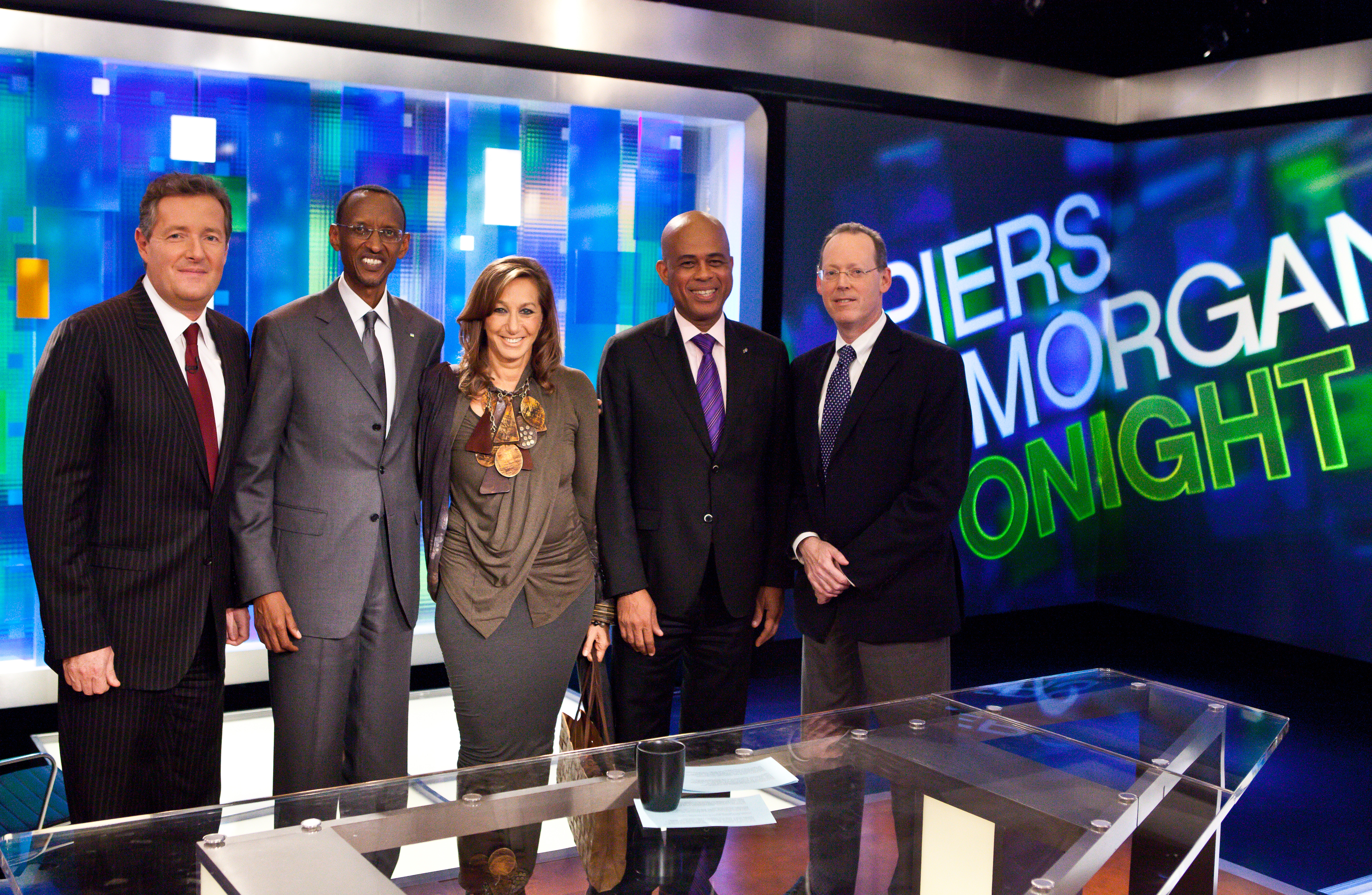In this image, five individuals are standing in a line, posing behind a large, clear rectangular glass table positioned on hardwood flooring. The setting appears to be a well-lit TV studio, with a prominent projected screen in the background displaying the words "Piers Morgan Tonight." The individuals are centralized in the image and are all dressed in formal attire. 

On the left stands Piers Morgan, identifiable by his black suit, white shirt, and red tie, smiling confidently. Next to him, a thin man with darker skin wears a gray suit. The woman in the center sports a brown top, a gray skirt, a scarf, long wavy dark brown hair, and a big, chunky necklace. To her right is another man with darker skin, dressed in a black suit and purple tie. At the far right, a Caucasian man with short hair, glasses, a dark blue jacket, a blue tie, and brown pants completes the lineup. 

The background features shades of blue and white lights, emphasizing the dynamic studio ambiance. The entire scene, bathed in a variety of colors including black, white, green, blue, yellow, gray, purple, and red, highlights the professional and engaging atmosphere of the set.